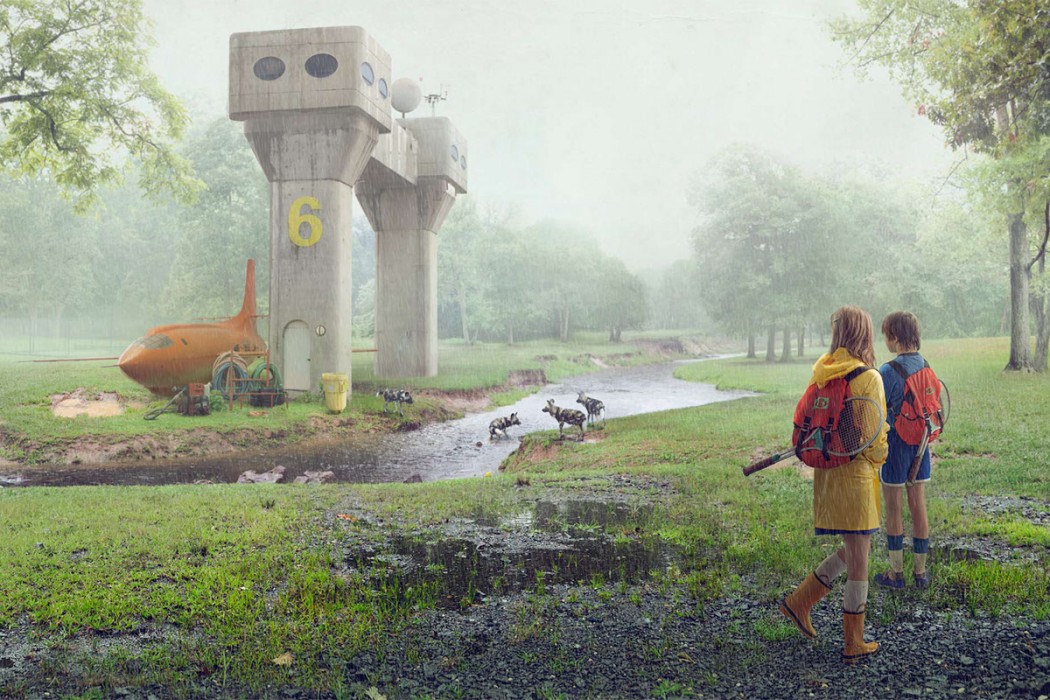In this detailed and realistic painting, we see a rainy, foggy scene featuring two children exploring near a river. The girl, closest to the camera, wears a yellow raincoat and matching yellow rain boots over knee-high white socks. She carries a red backpack with a tennis racket protruding from it. The boy, slightly further back, is dressed in a blue shirt, blue shorts with white trim, blue and white socks, and blue sneakers, also carrying a similar red backpack with a tennis racket. 

The background showcases a misty white sky and a gray river surrounded by greenery. To the left, a green tree stands prominently. Near the river, a group of indistinct animals, possibly hyenas or wild dogs, drink from the water. 

Prominently positioned is a concrete structure with two towers joined at the top, featuring oval-shaped windows and an arched white door facing the camera. The structure is marked with a yellow number 6. Beside it, an aged orange airplane rests near some equipment, including hoses and buckets, adding to the scene's eclectic and mysterious atmosphere. The artist has skillfully depicted the rain and its impact on the scene, with visible raindrops hitting the river's surface, enhancing the painting's lifelike quality.